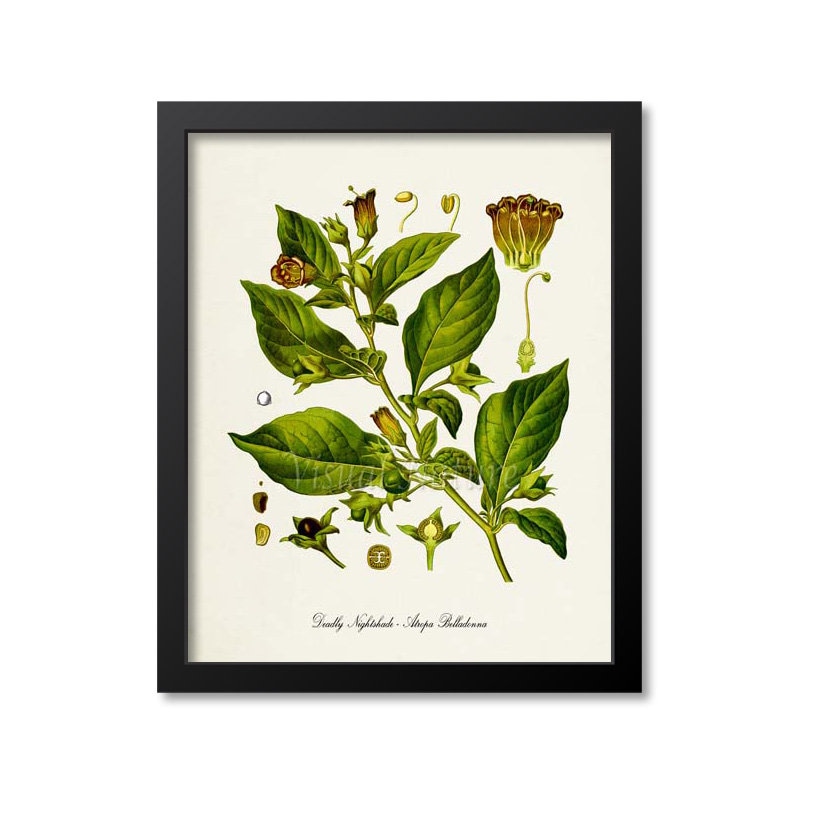This framed artwork depicts a detailed botanical illustration of a plant cutting, showcased in a very thin, pure black frame against a white background. The central image features a single branch with six large, roughly oval-shaped leaves and a few smaller leaves, all of which are green with prominent veins. Surrounding the main illustration are several smaller pictures that provide close-up views, including a cross-section of one of the flowers in the upper right corner and illustrations of both ripe and unripe berries in the lower left corner. The plant is adorned with flowers in various stages of growth; the mature flowers are brownish with rusty-red accents and appear somewhat frail and old, while the emerging flowers are greener with spherical bases. Some small green berries can also be seen on the plant. Stylized cursive script is present at the bottom of the illustration, presumably noting the plant's name, although it is too small to be legible. This intricate artwork, with its detailed botanical elements and naturalistic dead and blooming flowers, would likely appeal to someone with a keen interest in gardening or plant identification.